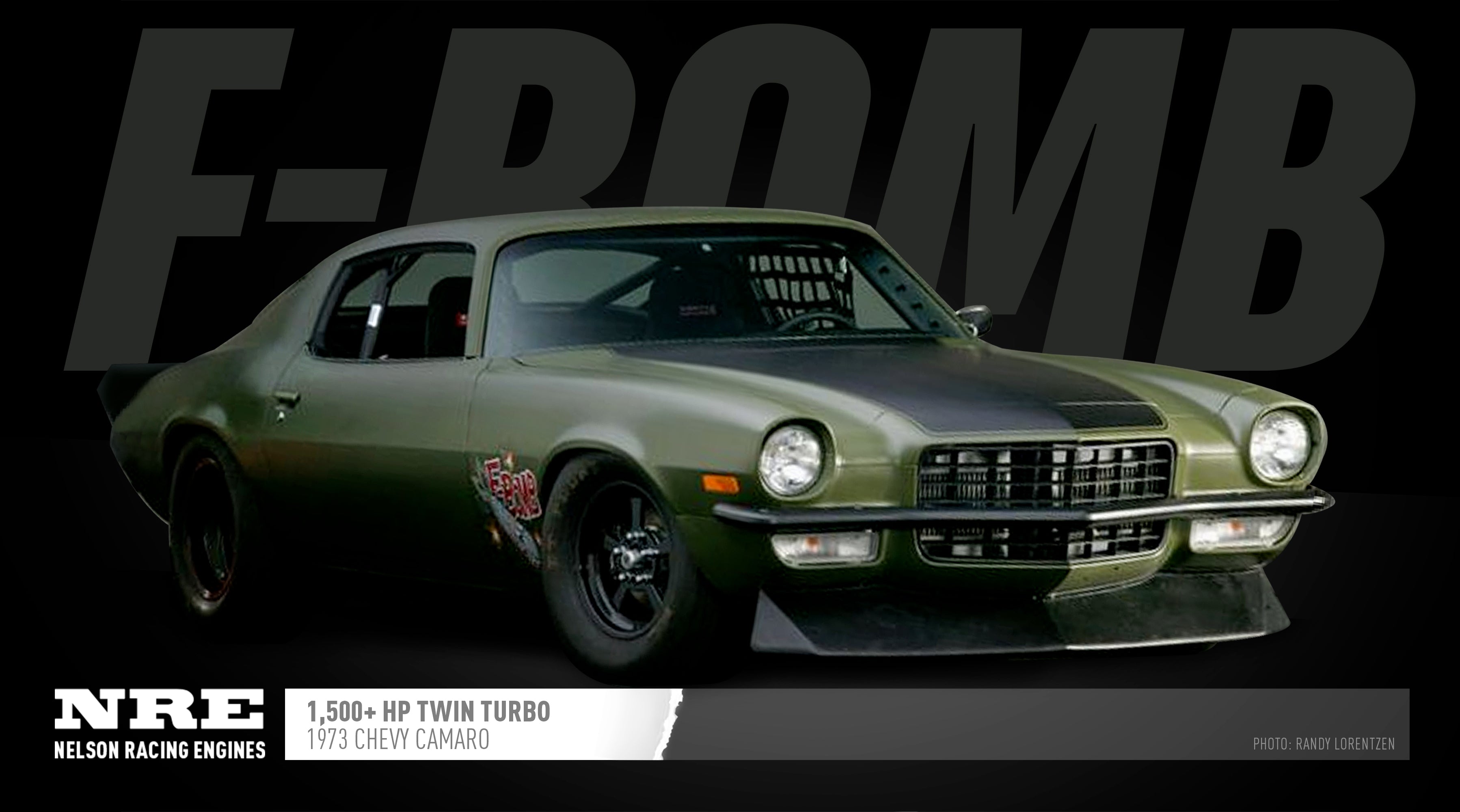This photograph, captured by Randy Lorentzen, features a 1973 Chevy Camaro positioned at a three-quarter angle facing right. The iconic two-door sports coupe displays a striking green exterior with a distinctive black center stripe on the hood, transitioning to a darker green along the bottom side of the passenger door and a lighter green on the top. The car boasts a black front grille with rectangular and gray details, round headlights, and a signature chrome bumper representative of early 1970s Camaro design. The rear of the car includes a wing and the windows are open, revealing a net above the steering wheel, suggesting its use as a race car. The background is a very dark gray with prominent light gray text that reads "F-Bomb." Below the car, a horizontal bar is divided into sections, with white text on a black background reading "NRE" followed by "Nelson Racing Engines," and a white section with text "1500 plus HP Twin Turbo." The final section in light gray text reads "1973 Chevy Camaro." The photograph's details are completed by the mention of a note in the bottom right corner, crediting Randy Lorentzen as the photographer.